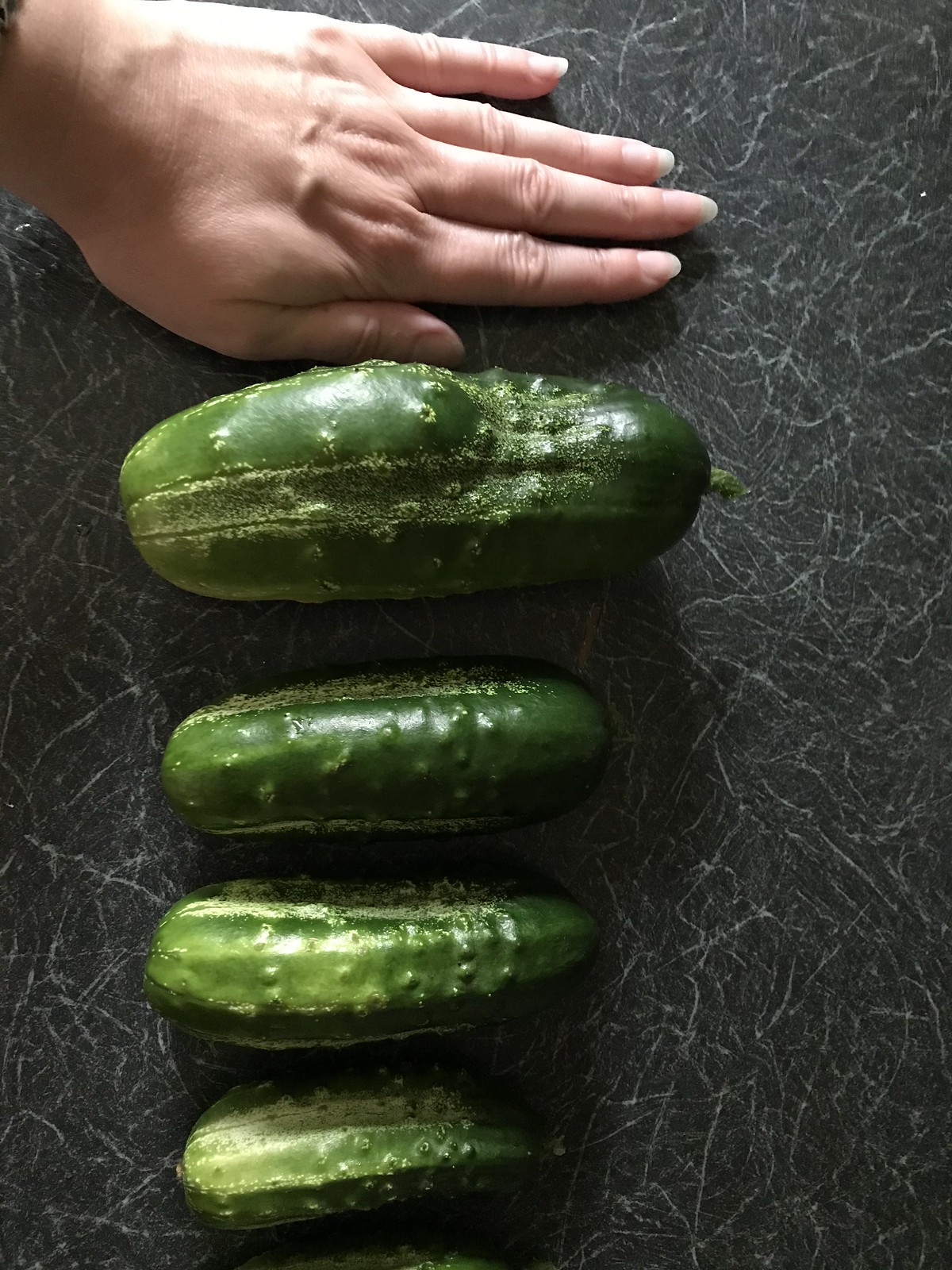This is a photograph showing four cucumbers of varying sizes lined up on a dark gray, leather-like surface that features a scratched white veining pattern. The smallest cucumber is at the bottom, with each subsequent cucumber increasing in size; the second from the top is nearly the same size as the one below it, while the largest cucumber at the top is thicker and somewhat lumpy. Above this largest cucumber, a left hand, with long, manicured nails and no polish, is placed flat against the surface for size comparison. The hand is positioned with the thumb pointing downward, showing that the biggest cucumber is approximately the same length as the hand from the middle finger to the wrist. The cucumbers are short and stubby, resembling those commonly used for pickling. The entire arrangement appears meticulously organized to demonstrate the relative sizes of the cucumbers.